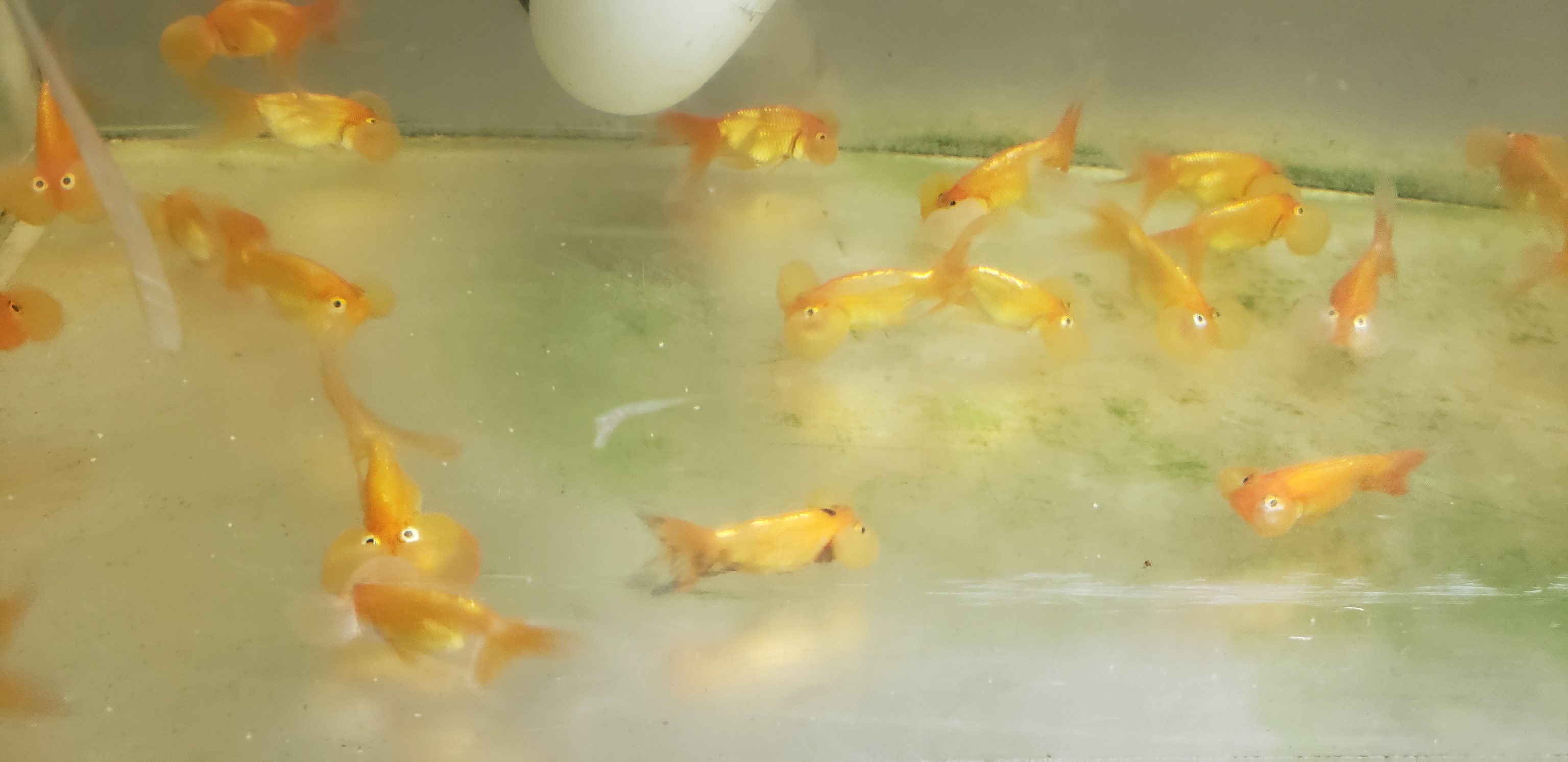The image showcases a close-up view of a fish tank containing a vibrant collection of small, yellow-orange fish that resemble but are not goldfish. These fish have distinctively amusing, large, googly eyes positioned on top of their heads, giving them a comical appearance. There are more than a dozen of these tiny, immature fish scattered throughout the clear water of the tank. Notably, the tank also contains an object in the top center, likely a pump or filtration device, which is partially visible and situated at the back. A strip-like outline is faintly visible on the top left, presumably part of the tank setup. The clear water shows some green splotches, hinting at the presence of algae, adding to the naturalistic details of the scene.